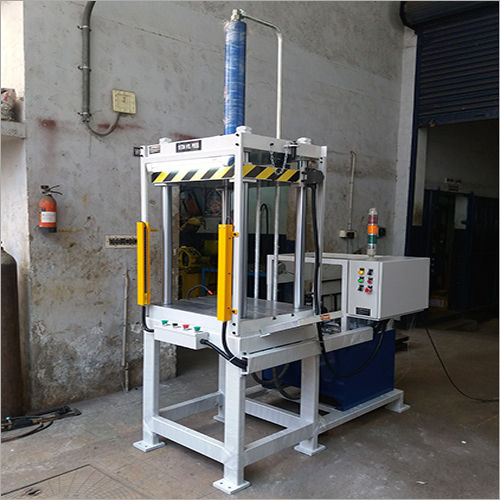The image captures a detailed side-angle view of a large industrial machine situated in what appears to be a warehouse or factory environment with concrete floors and walls. The machine, positioned centrally and at a diagonal, is anchored on a white hollowed square base and has a prominent blue cylinder at the top wrapped in plastic. This cylinder is attached to a yellow and black caution-striped section beneath it. Below, the front-facing control panel features four buttons colored green, black, red, and green, respectively. On the machine's right-hand side, there is a tall grated blue door that opens further into the warehouse. Adjacent to the machine, on the left wall, a mini fire extinguisher is mounted.

The rear section of the machine resembles a rectangular microwave-like structure with a cylindrical component on top displaying an array of colored andons in red, yellow, and green. The control interface on this segment includes six buttons (yellow, black, green, red, black, and red) and a rectangular black button situated above a blue cube. The setting behind the equipment features a partially opened blue or black garage door on the back right, allowing a glimpse of the broader warehouse area. Various colors such as blue, yellow, black, white, gray, and brown are visible throughout the image, adding to the detailed industrial ambiance.